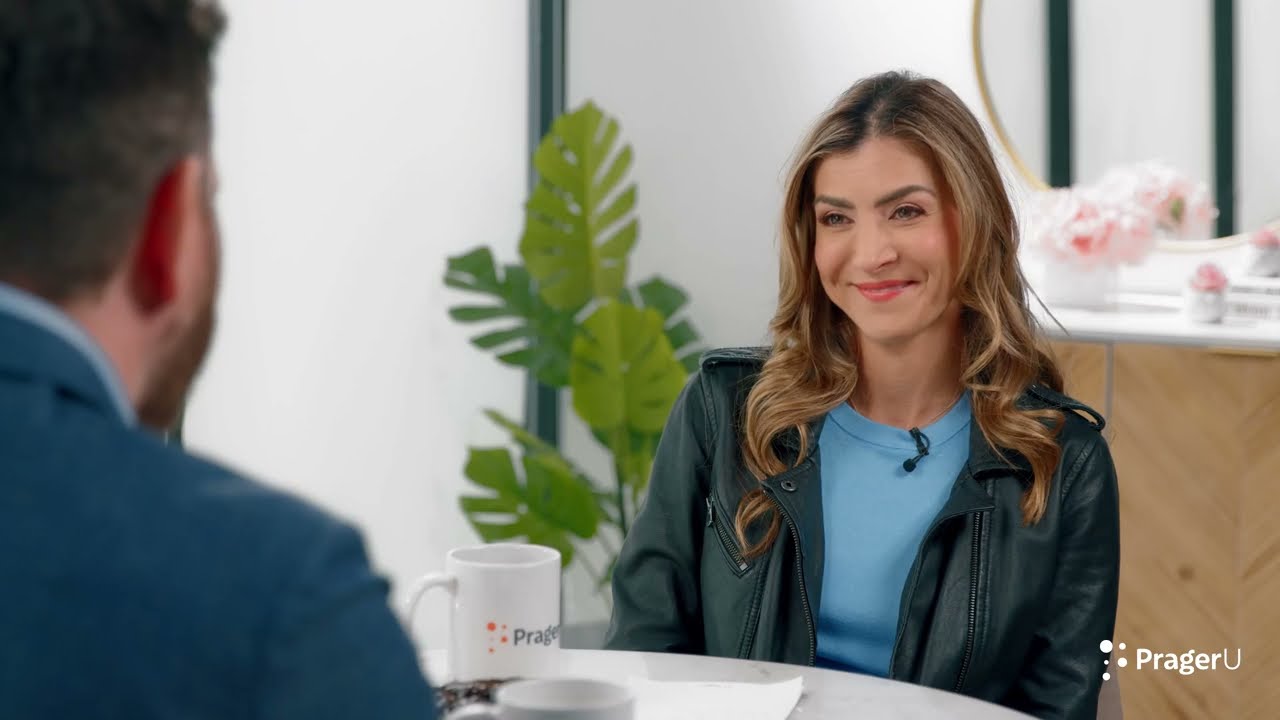In this image, which appears to be a promotional photograph for PragerU, the focal point is a woman and a man sitting at a round white table engaged in what seems like a meeting. In the center of the table, there is a white coffee cup emblazoned with the PragerU logo, featuring orange circular dots. The woman, positioned on the right side of the image, has medium blonde hair that cascades in curls just below her shoulders. She is wearing a blue shirt with a black leather jacket over it and has a clip-on microphone attached to her collar. Her expression is a slight, forced smirk, and she has rosy lips, dark eyes, and dark eyebrows. The man, slightly out of focus and to the left, is facing away from the camera towards the woman. He has short brown hair, a beard, and is clad in a dark blue suit with a matching dress shirt. Both individuals are Caucasian.

The background features a white wall and a lush banana leaf plant with large green leaves positioned centrally behind the woman. To her right, past the plant, there is a light brown cupboard topped with a marble-like surface, adorned with light pink flowers, contributing to the decorative ambiance. Above the cupboard, a circular mirror is mounted on the wall. In the lower right corner of the image, the PragerU logo is prominently visible, reinforcing the brand's presence in the photograph.